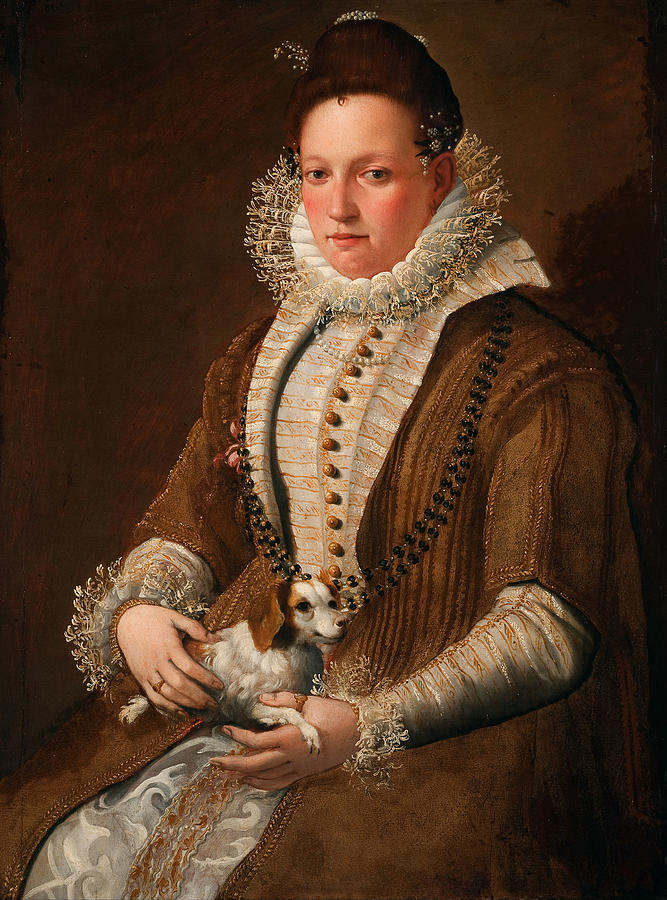The image is a detailed oil painting from the Renaissance or Elizabethan era, depicting an androgynous figure with soft cheeks, short hair, and an elaborate, layered, full-body brown outfit that extends past their knees. They are adorned with large necklaces, including one made of pearls, and their hands, which have two ringed fingers and are draped in long sleeves, are resting on their lap, holding a tiny white dog with brown ears. The subject appears to be seated and gazing directly at the viewer. The background is a solid brown color, accentuating the intricate details of their attire, which includes copper or bronze buttons and a headpiece with brown fabric and floral sprigs. The collar around their neck is decorative, featuring sprigs of white, further suggesting a sense of high status or royalty.